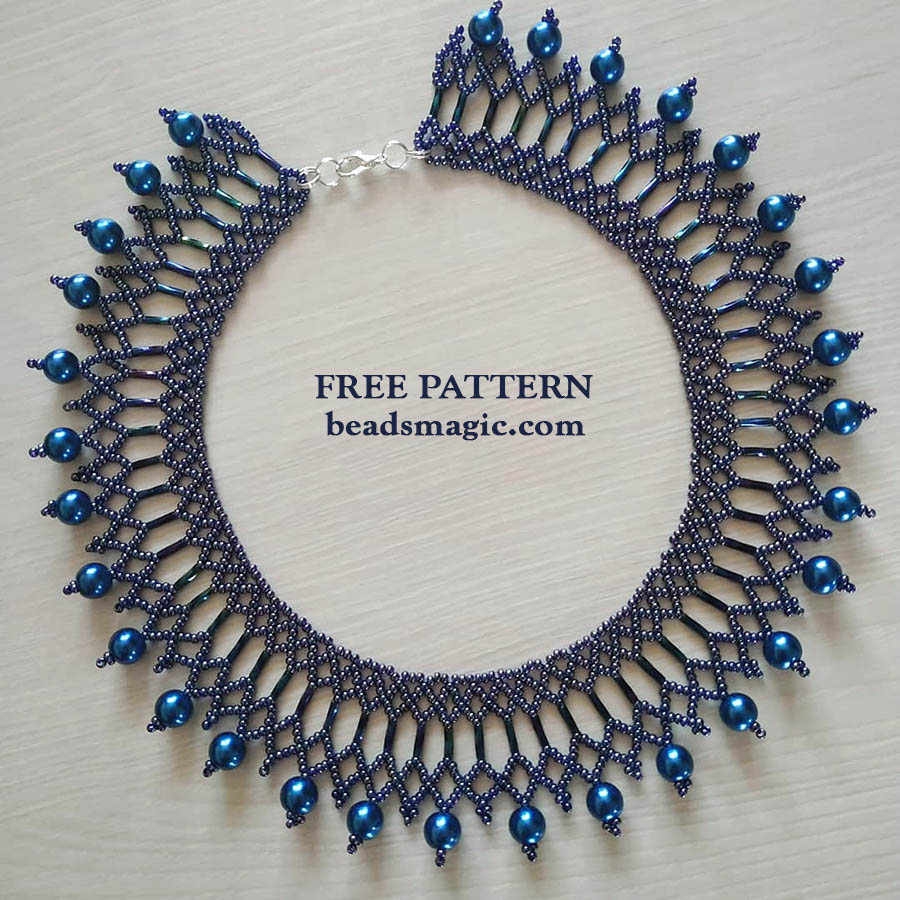This detailed image showcases a finely crafted beaded necklace, featured against a gray background, potentially set on a table. The necklace appears to be suited for a small shop or Etsy shop, as it has a professional and clear photograph quality. It could also serve as an advertisement for the free pattern available on beadsmagic.com, as indicated prominently in the center of the image. The necklace is an intricately designed piece, possibly of native craftsmanship, with a blend of blue, black, and purplish beads. 

This choker-style necklace forms a perfect circle, secured by a silver clasp, designed to fit snugly around the neck. The beadwork consists of multiple levels: the innermost layer features small diamond-shaped tiny beads, followed by elongated tube-like beads. The outer layer consists of medium-sized blue glossy beads, some resembling pearls, which hang down to create a sophisticated, multi-dimensional effect. This elegant design, with its textural interplay of very tiny gunmetal gray beads, cylindrical beads, and larger blue circular beads, offers a free pattern that can be recreated by beading enthusiasts.